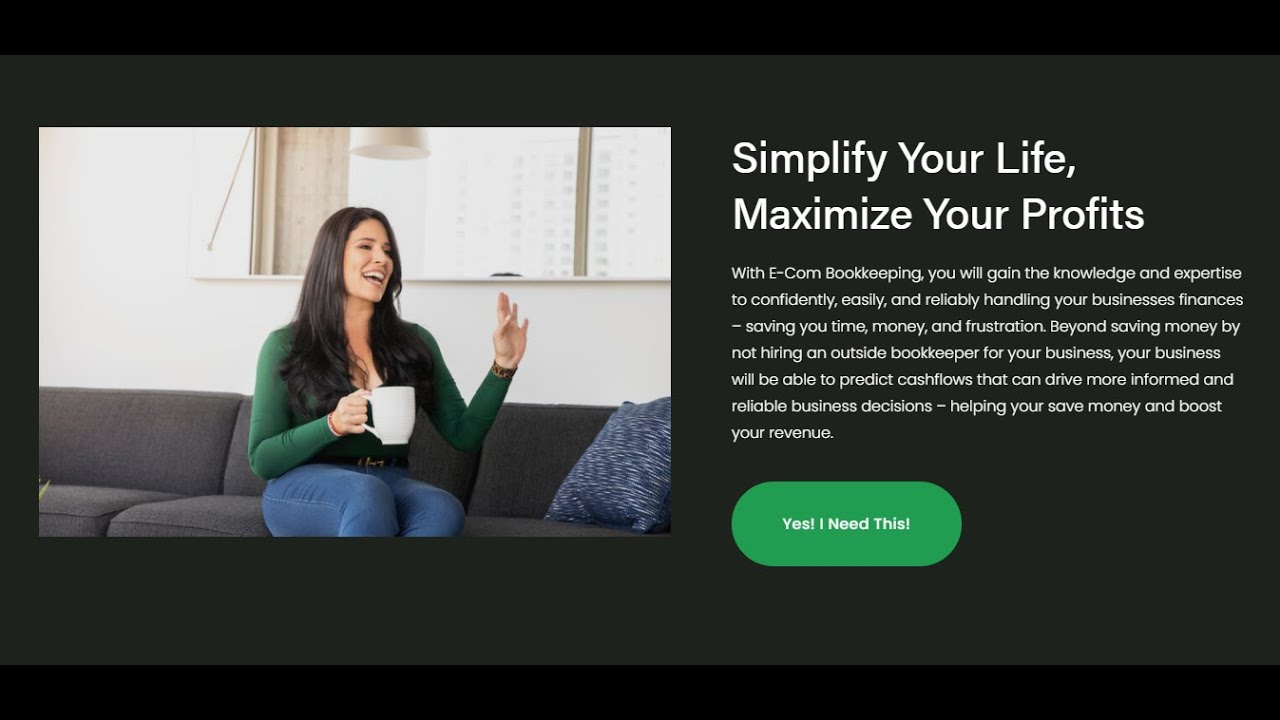In this captivating image, a page prominently displays the message "Simplify Your Life, Maximize Your Profits." The text describes the benefits of e-commerce bookkeeping, stating that it provides the knowledge and expertise to confidently, easily, and reliably manage business finances. This service is portrayed as a means to save time, money, and frustration, allowing businesses to avoid the costs of hiring an external bookkeeper and instead harness accurate cash flow predictions for more informed and reliable business decisions, ultimately boosting revenue. 

The text, written in white, is set against a striking green badge. To the left of the page, a woman clad in blue pants and a green top is seen holding a cup of coffee while seated on a couch. She appears to be joyfully engaging in a conversation, her cheerful demeanor adding a lively touch to the composition. The overall background is predominantly black, which serves to highlight the vibrant colors and dynamic elements within the image.